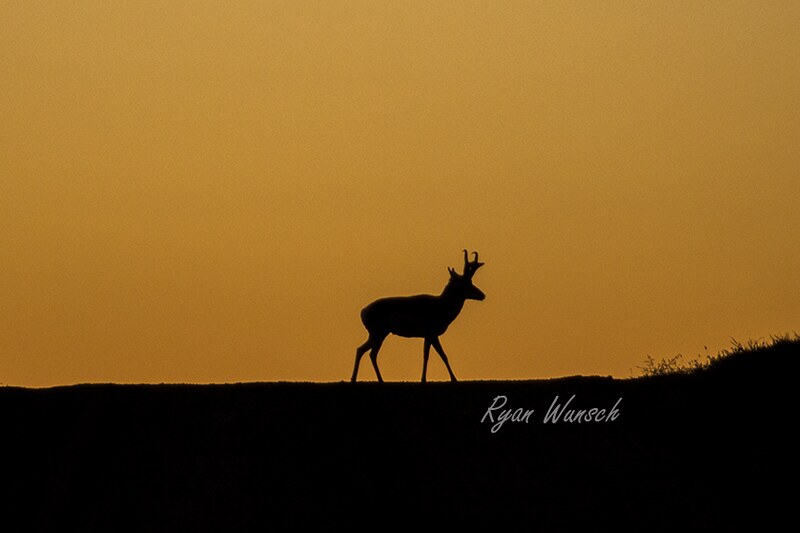The image captures a serene and striking sunset scene with an orange-golden sky, where a setting sun casts a warm glow across the horizon. Dominating the foreground, a lone reindeer, discernible only by its dark silhouette, strides purposefully to the right atop a low hill lined with sparse grass. Its antlers are visible against the glowing backdrop, adding a touch of detail to the shadowy figure. The ground, a dark black, forms a solid contrast against the luminous sky, which is painted in unparalleled hues of orange and gold. The entire composition is framed horizontally like a rectangle, enhancing its panoramic feel. The photograph, signed by Ryan Wunsch in elegant script, captures the stillness and beauty of the moment with an almost ethereal quality.